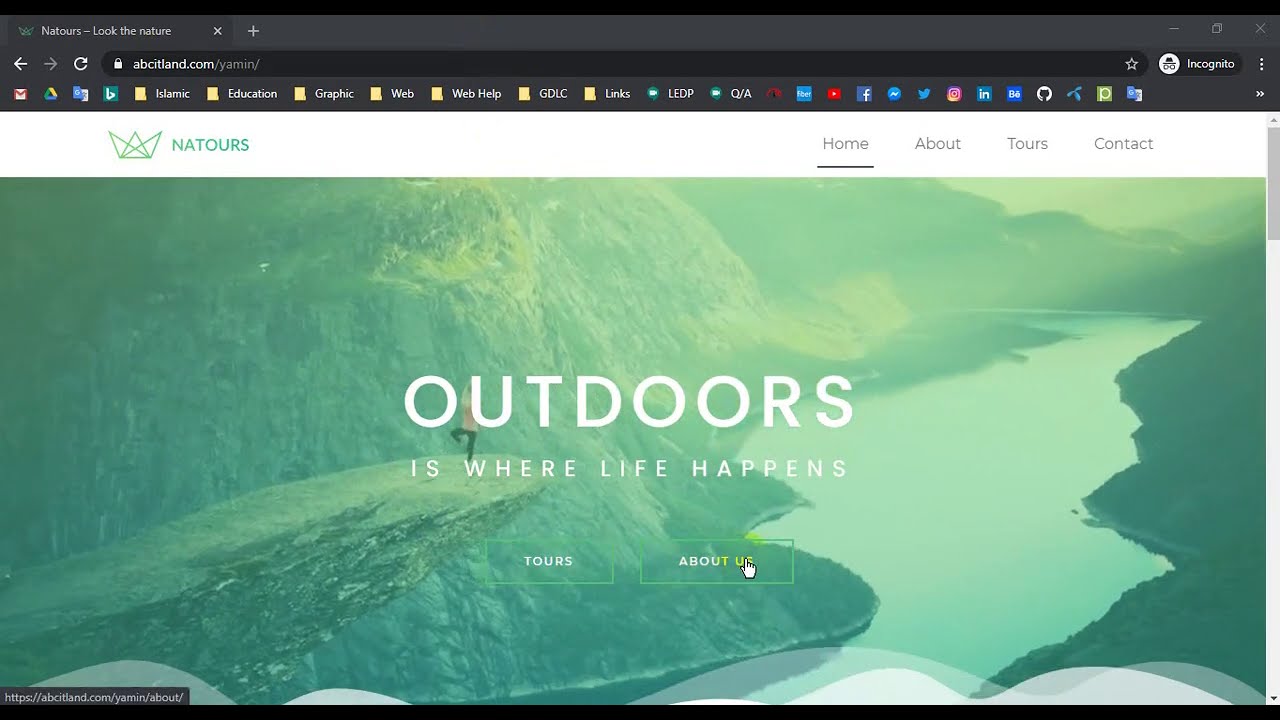The image features a prominent black header at the top, containing small, unreadable text followed by various icons, symbols, and arrows including an 'X', a plus mark, left and right arrows, backup arrows, and a search box. Beneath these icons, there are labels for 'News,' 'Education,' 'Graphic,' 'Web Help,' as well as categories like 'Links,' 'LEDP,' and 'Q4s.' The header also includes recognizable social media icons such as Facebook.

Below the header is a spacious white area displaying a small crown graphic alongside the text "Natures." The navigation menu beneath this includes underlined links: 'Home,' 'About,' 'Tours,' and 'Contact.'

The central focus of the image is a stunning large photograph of verdant, grassy hills and a serene lake winding through the landscape, captioned with the inspirational phrase "Outdoors is where life happens" in white text. 

Below this scenic photo, there are two interactive buttons labeled 'Tour' and 'About Us,' with a hand icon hovering over the 'About Us' button. In the bottom left corner of the image, a small white box contains an HTTPS address, beside a thin black line.